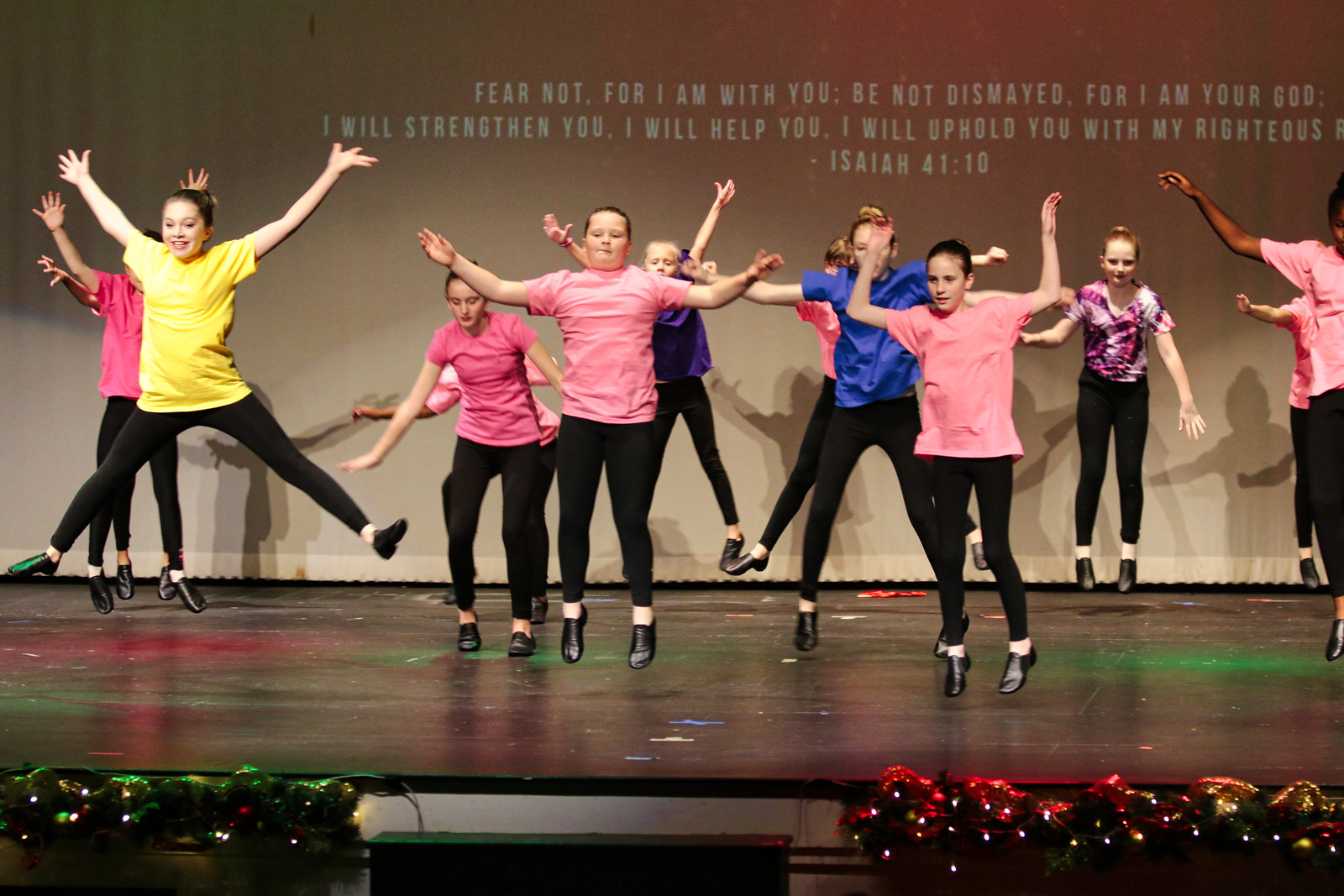In the photograph, a dynamic dance performance unfolds on a black stage, dramatically illuminated by red and green spotlights. The dancers, a group of young females, are all dressed in black spandex leggings and black shoes. Their vibrant t-shirts add bursts of color, with several in pink, one in yellow, two in blue, and another in tie-dye. Their hair is mostly pulled up and back, emphasizing a clean and energetic look as they leap and jump. Arms are outstretched and legs are either straight down or extended, capturing various stages of their jumps, though not all in perfect sync.

The backdrop is a white curtain, dimmed slightly by the lighting, featuring a projected text in white that reads, "Fear not, for I am with you. Be not dismayed, for I am your God. I will strengthen you, I will help you, I will uphold you with my righteous," followed by the partially cut-off citation, "Isaiah 41:10." Shadows of the dancers cast dramatically against this backdrop, adding depth to the scene.

In front of the stage, several decorative elements include what appear to be fluorescent lights in blue, red, and possibly gold hues. These elements create an additional layer of visual interest. The overall composition of the image harmonizes the vibrant energy of the dancers with the profound message projected behind them, creating a captivating and inspirational moment.